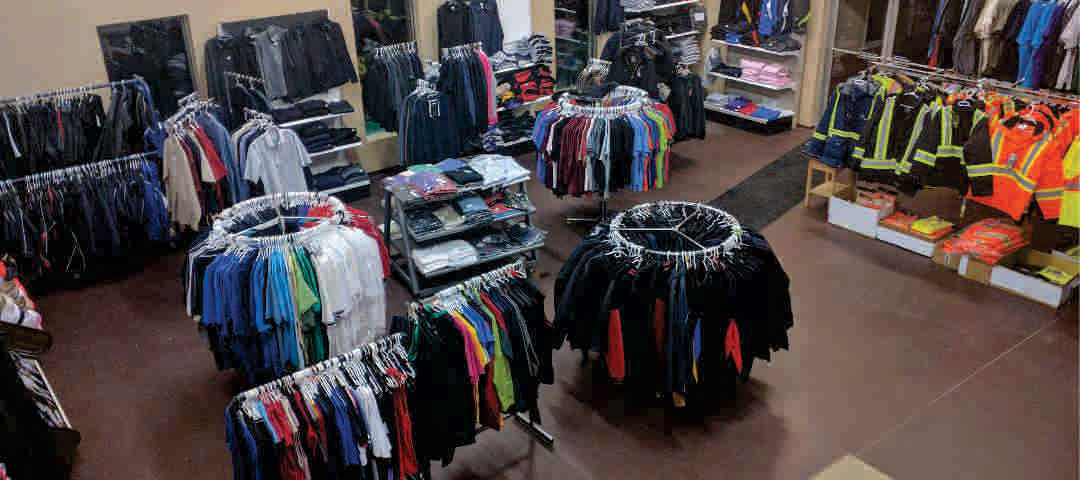This aerial image captures an interior shot of a men's clothing store, taken from a ceiling-mounted camera. The store layout is well-organized with several types of racks. Centrally, there are three circular racks predominantly filled with t-shirts; one rack features mainly darker shirts such as black, while another has lighter shades including white, blue, and red. Adjacent to these are two shorter racks, adding variety to the middle space. To the right, a section of jackets stands out, with eye-catching colors like orange, black, yellow, and blue, adorned with neon yellow and gray reflective stripes, indicative of safety or emergency wear. The jackets and other clothes on the racks display a wide spectrum of colors, including yellow, black, orange, white, brown, red, green, and blue. The back wall holds dark clothing items, with something pink visible on shelves. The store features a tan wall at the rear and a brown floor, accented by a black strip and a runner rug leading to a see-through door. The overall ambiance suggests a neat and functional men's clothing store, offering a diverse range of apparel from everyday t-shirts to specialized reflective jackets.